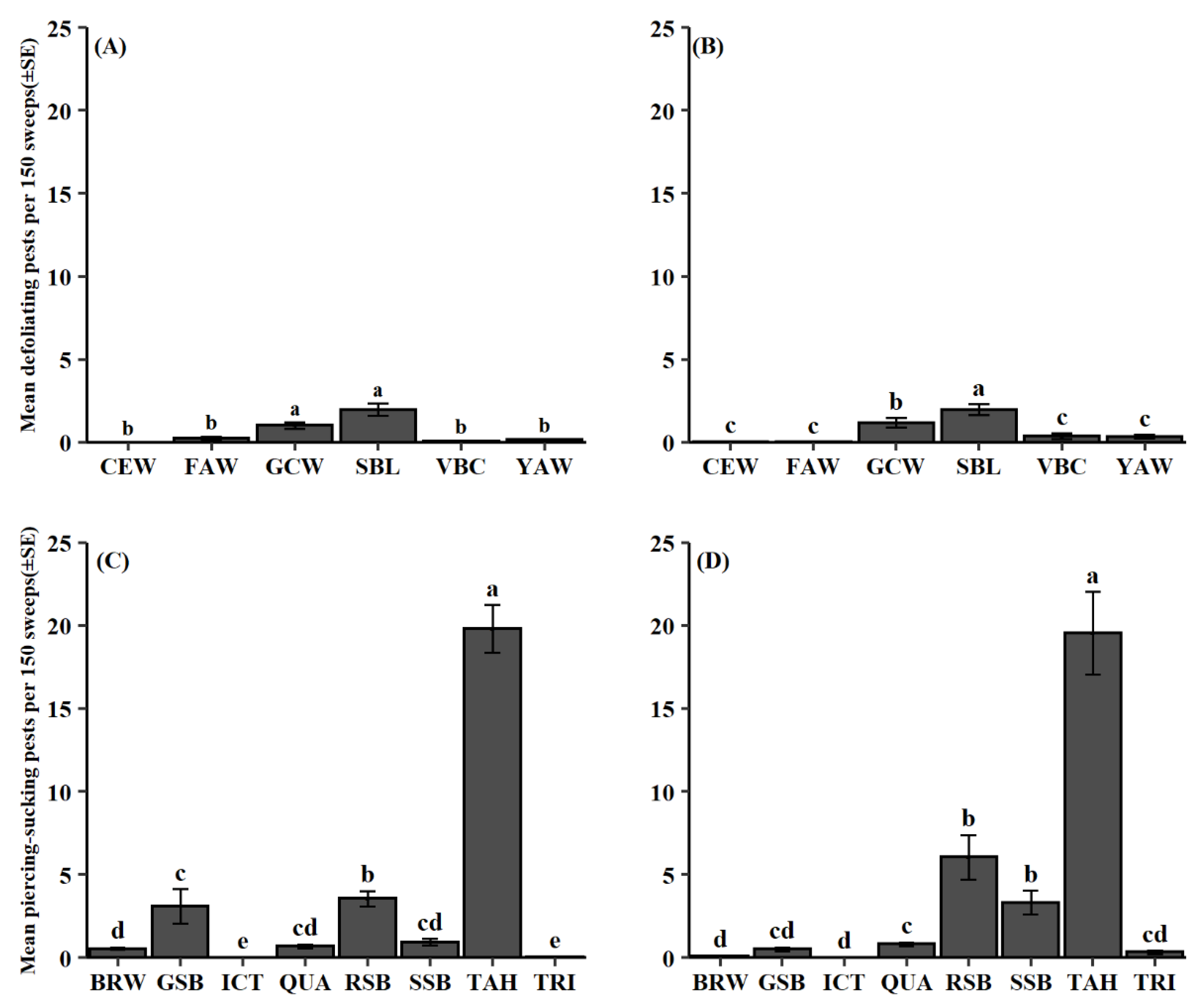The image depicts four black-and-white bar graphs arranged in a 2x2 grid. The top-left graph, labeled as Graph A, is titled "Mean Defoliating Pests per 150 Sweeps." It ranges vertically from 0 to 25 and horizontally includes categories CEW, FAW, GCW, SBL, VBC, and YAW. Both Graph A and the top-right graph (Graph B) exhibit a similar bell-shaped distribution pattern, with Graph B also ranging from 0 to 25 on the vertical axis and identical categories on the horizontal axis.

The bottom-left graph, labeled as Graph C, is titled "Mean Piercing-Suckling Pests per 150 Sweeps." It shares its vertical axis scale of 0 to 25 with Graph D, the bottom-right graph. These two graphs, C and D, feature the categories BRW, GSB, ICT, QUA, RSB, SSB, TAH, and TRI along the horizontal axis. Notably, both Graph C and Graph D show significantly higher bars at the category TAH compared to the other categories, indicating a much denser presence of pests in this group.

Overall, the image contrasts the relatively minimal data points and bell-shaped distributions of the top graphs with the pronounced, higher bars of the bottom graphs, especially under the TAH category.